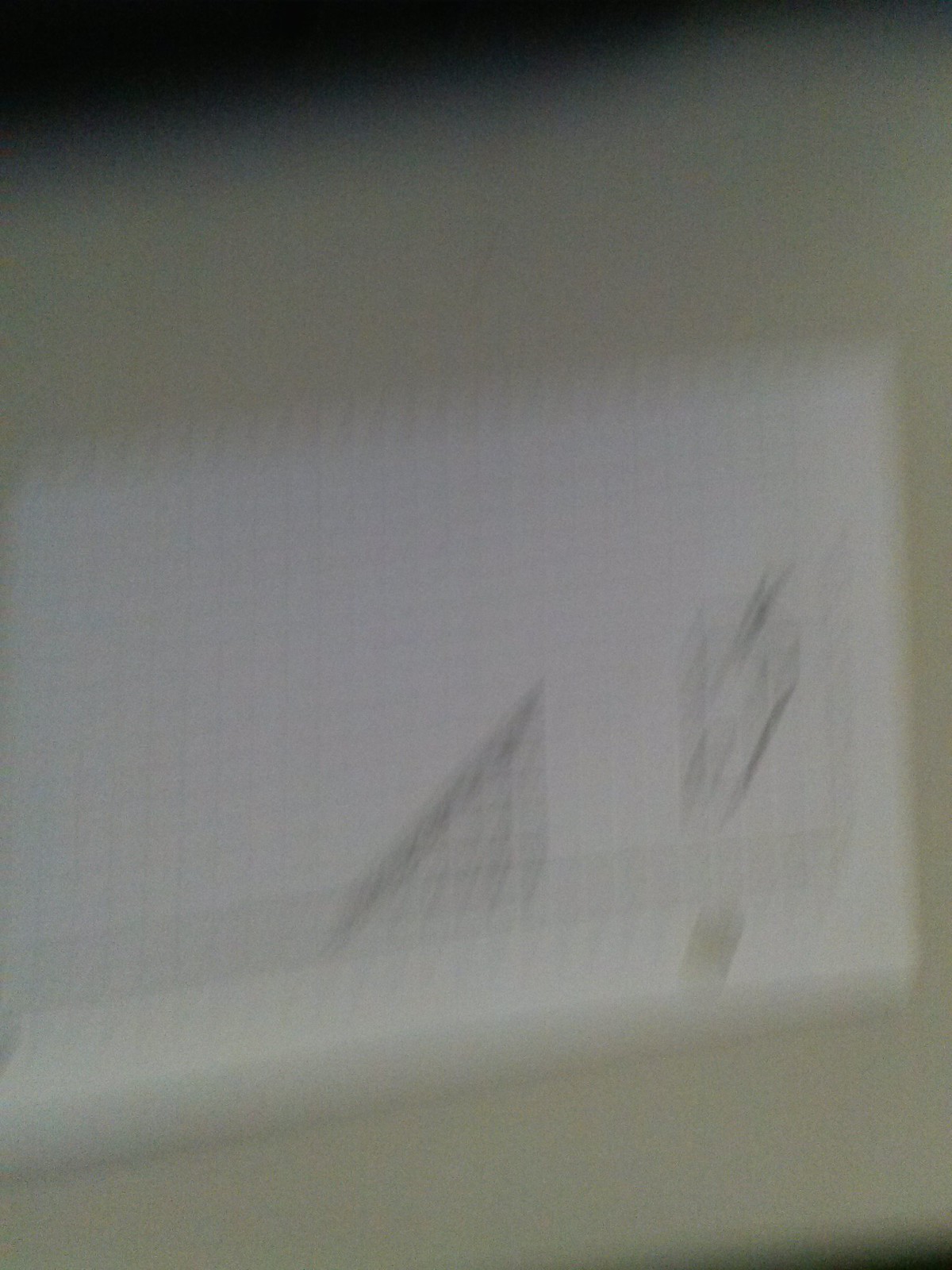A slightly blurry and out-of-focus image captures a tabletop with a spiral-bound notebook lying open on its surface. The notebook contains grid paper featuring a variety of rudimentary pencil sketches and geometric shapes. Dominating the page is a horizontally shaded parallel stripe intersected by several diagonal lines. At the top right of the paper, a steeply angled, three-dimensional ramp is drawn, with the ramp's surface noticeably shaded darker than the rest. A smudge is visible at the bottom right corner of the paper, and next to the ramp, there is an indistinct geometric shape, adding to the assortment of basic sketches.